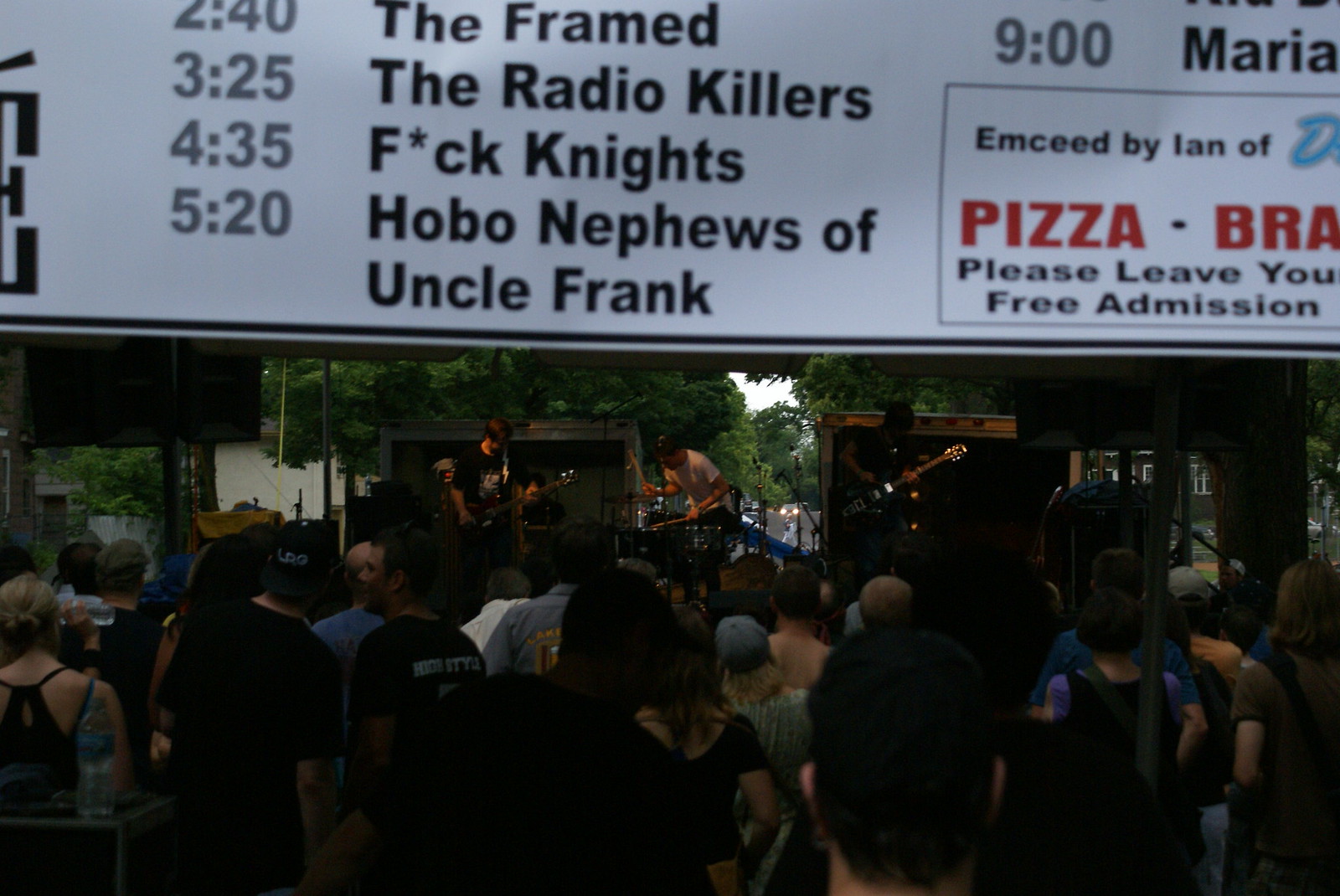The image is a detailed photograph of a live outdoor music show taken from the perspective of an audience member during the daytime. The foreground features a white banner spanning the top of the image and descending about an inch and a half from the top. This banner lists band schedules in light gray times and black titles: "2:40 - The Framed," "3:25 - The Radio Killers," "4:35 - F*ck Nights," and "5:20 - The Hobo Nephews of Uncle Frank." On the right-hand side of the banner, in red print, it mentions they have pizza and includes a cut-off line reading "emceed by Ian of…". Below the banner, the image captures a decent-sized crowd with their backs turned towards the camera, all facing a makeshift stage, which is set against a backdrop of a tree-lined street. On the stage are three band members bathed in shade, making them difficult to see clearly: two guitarists on either side and a drummer positioned in the middle. The overall ambiance suggests a laid-back, community-driven event.